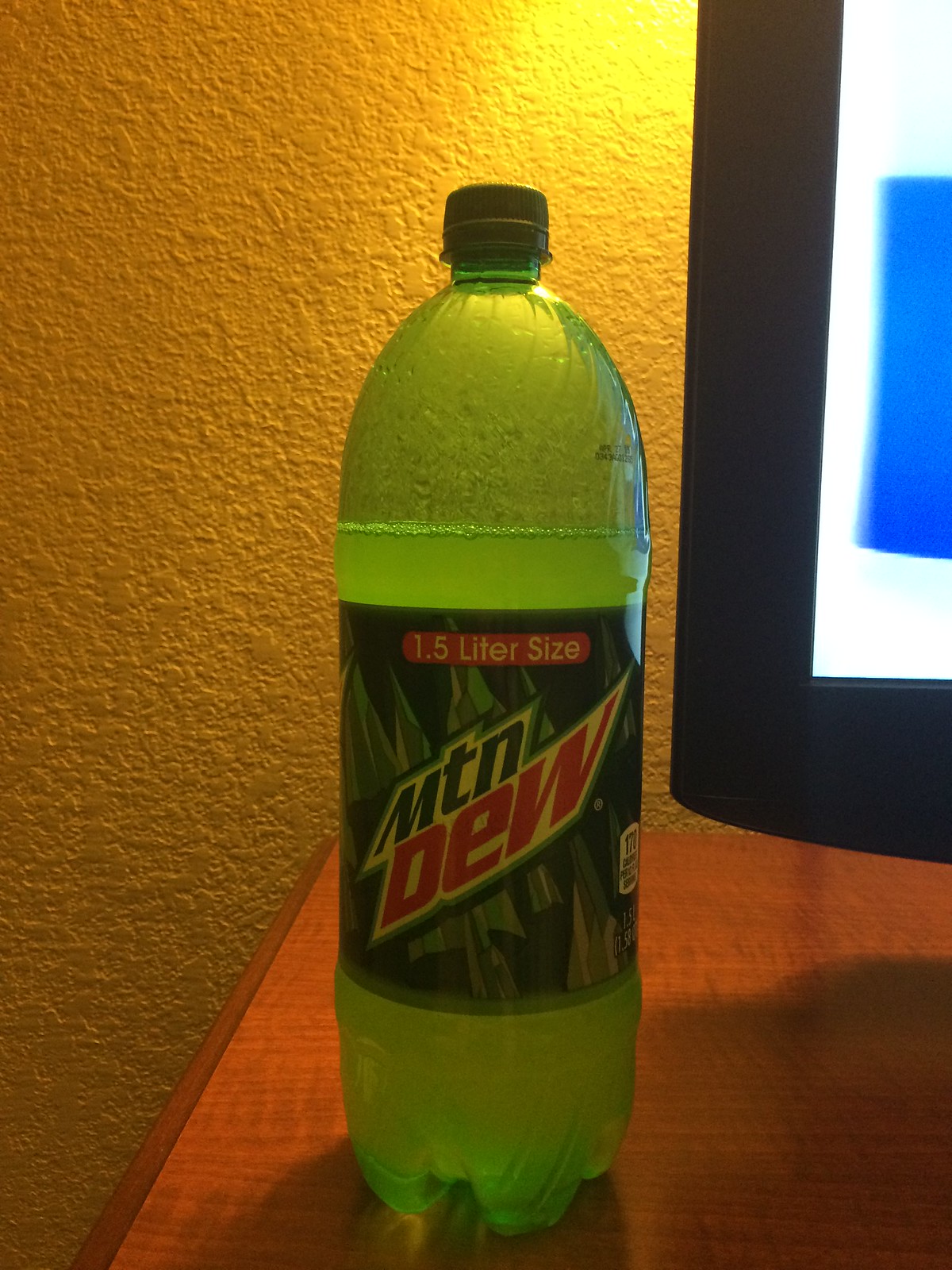Indoor photograph featuring an opened 1.5-liter bottle of Mountain Dew positioned on a dark cherry wood dresser or TV stand. The bottle is mostly empty, with only about half an inch to an inch of the neon green liquid remaining above the label. The label prominently displays the Mountain Dew logo and indicates 170 calories per serving on the bottom right. The off-white wall in the background appears yellowish under artificial lighting and has a textured surface. Adjacent to the bottle, on the right, is a TV or computer monitor.